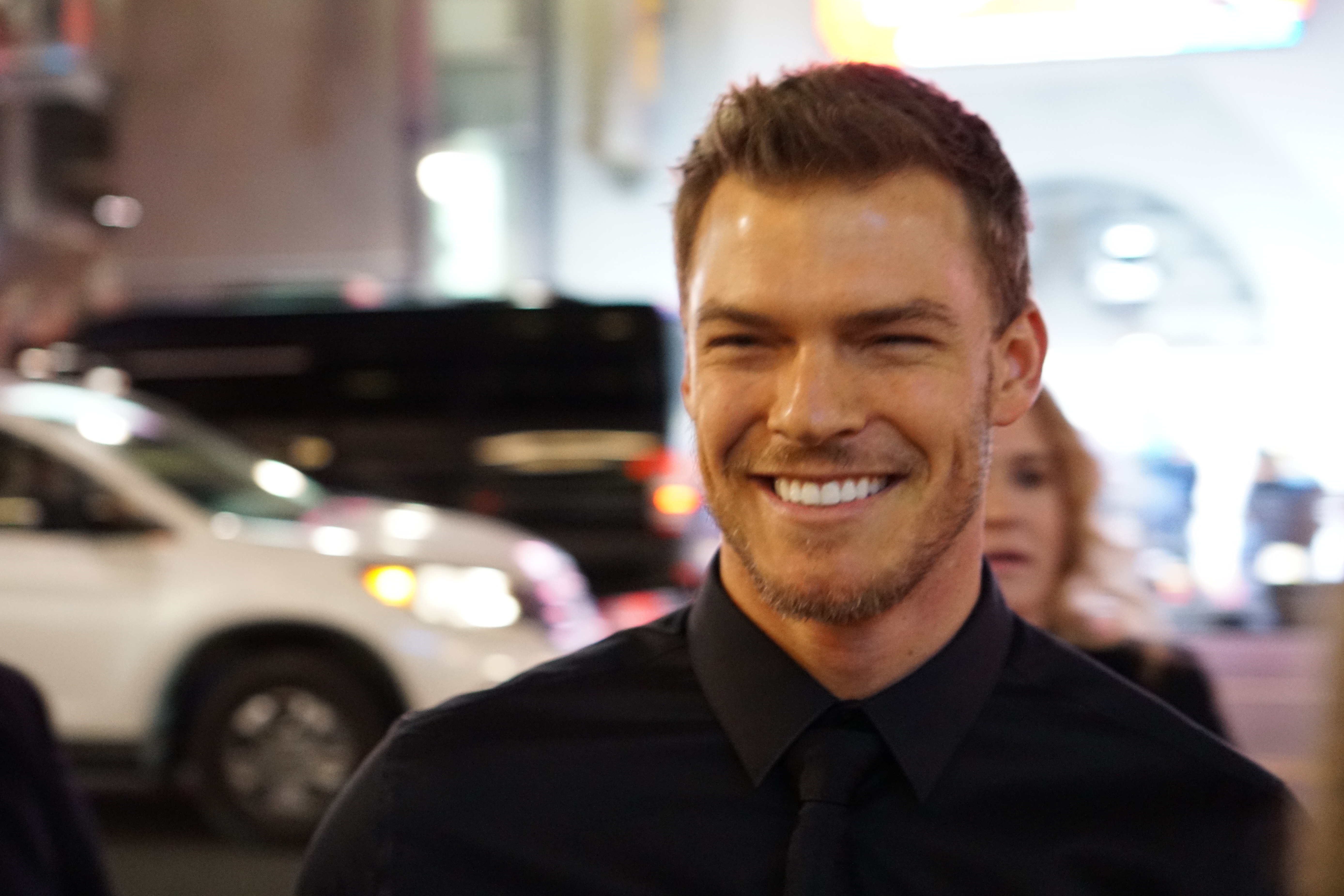This is a photograph, likely of actor Alan Ritchson, who is standing outdoors. He is smiling broadly, revealing his very white teeth, and is looking slightly off to the side rather than directly at the camera. His light brown hair is styled in a short, slightly spiky look. Alan is wearing a black shirt with a black collar and a black tie, but the image is zoomed in so only his face, his stubbly facial hair, and his shoulders are clearly visible. 

In the background, which is considerably blurred to keep the focus on Alan, a woman with blonde hair is partially visible, though her face is also blurry. She seems to be wearing a black shirt. Additionally, there is a white crossover SUV with golden-white headlights and black tires to the left of Alan, with potentially another dark, indistinct vehicle further behind it. The background colors include shades of black, white, and light blue, adding to the outdoor setting's mosaic effect. The overall composition emphasizes Alan's movie-star appearance and charismatic smile against the vaguely detailed backdrop.